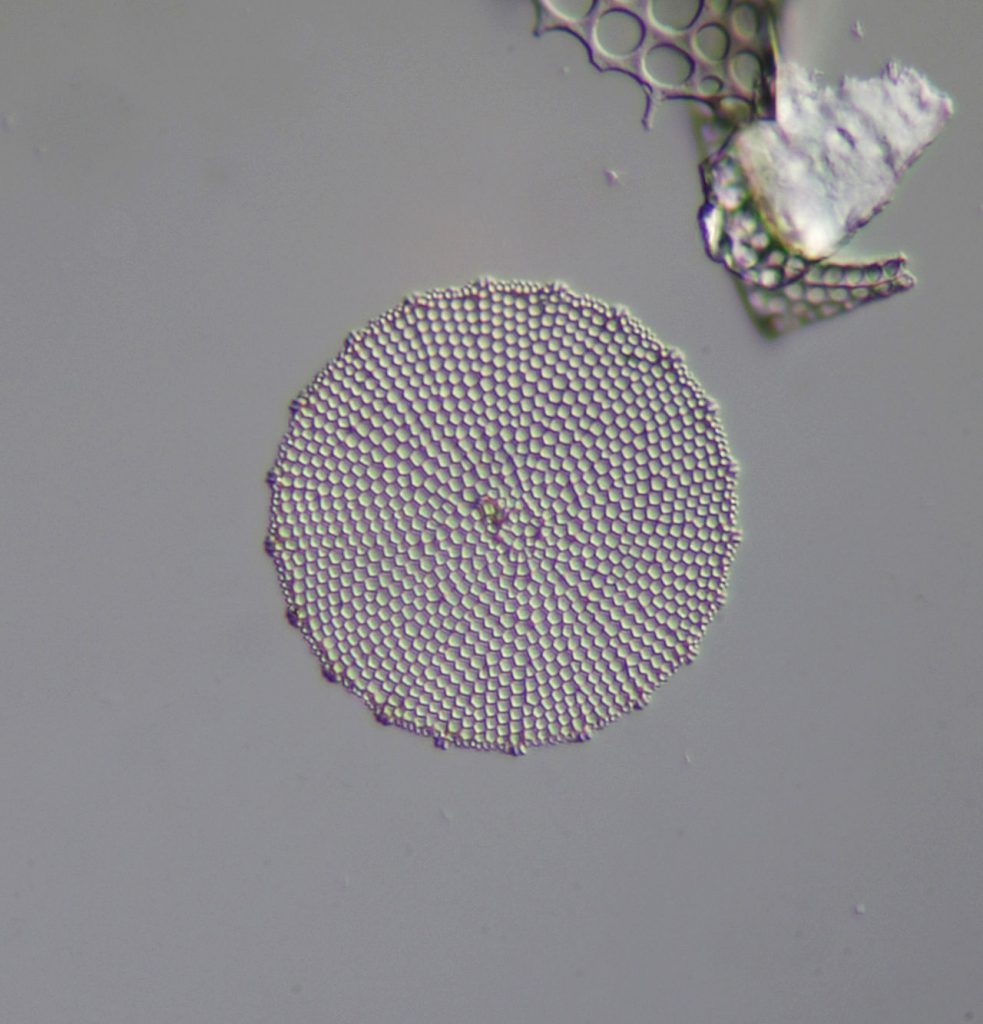The image appears to be a highly magnified, color photograph that resembles a microscopic view. Central to the picture is a circular, lily pad-like structure with a light purple hue, adorned with small white scales or dots, which gives it a textured appearance. This structure appears to have a raised rim and radiates a pattern of tiny circles towards its center. The background of the image is a dark gray, providing a stark contrast to the central feature. In the upper right quadrant, there is a secondary element, resembling shed skin or a wing-like structure with holes in it, also purplish in color, coupled with a small triangular pile of what appears to be white powder. This secondary element further emphasizes the microscopic nature of the image.